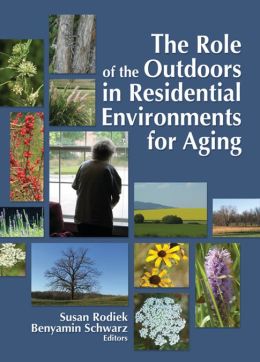The book cover, predominantly in shades of blue and teal, features the title "The Role of the Outdoors in Residential Environments for Aging" in prominent white text. The bottom of the cover lists the editors: Susan Brodick and Benjamin Schwartz. The design is adorned with various natural elements, including vibrant green leaves, red florals, brown tree bark, and both yellow and purple flowers. A central image captures an older woman with gray hair wearing a short-sleeved shirt and pants, gazing out of a window. She looks towards a landscape that includes rolling green hills, a partly clear sky, and bare tree trunks, suggesting a peaceful, natural environment.